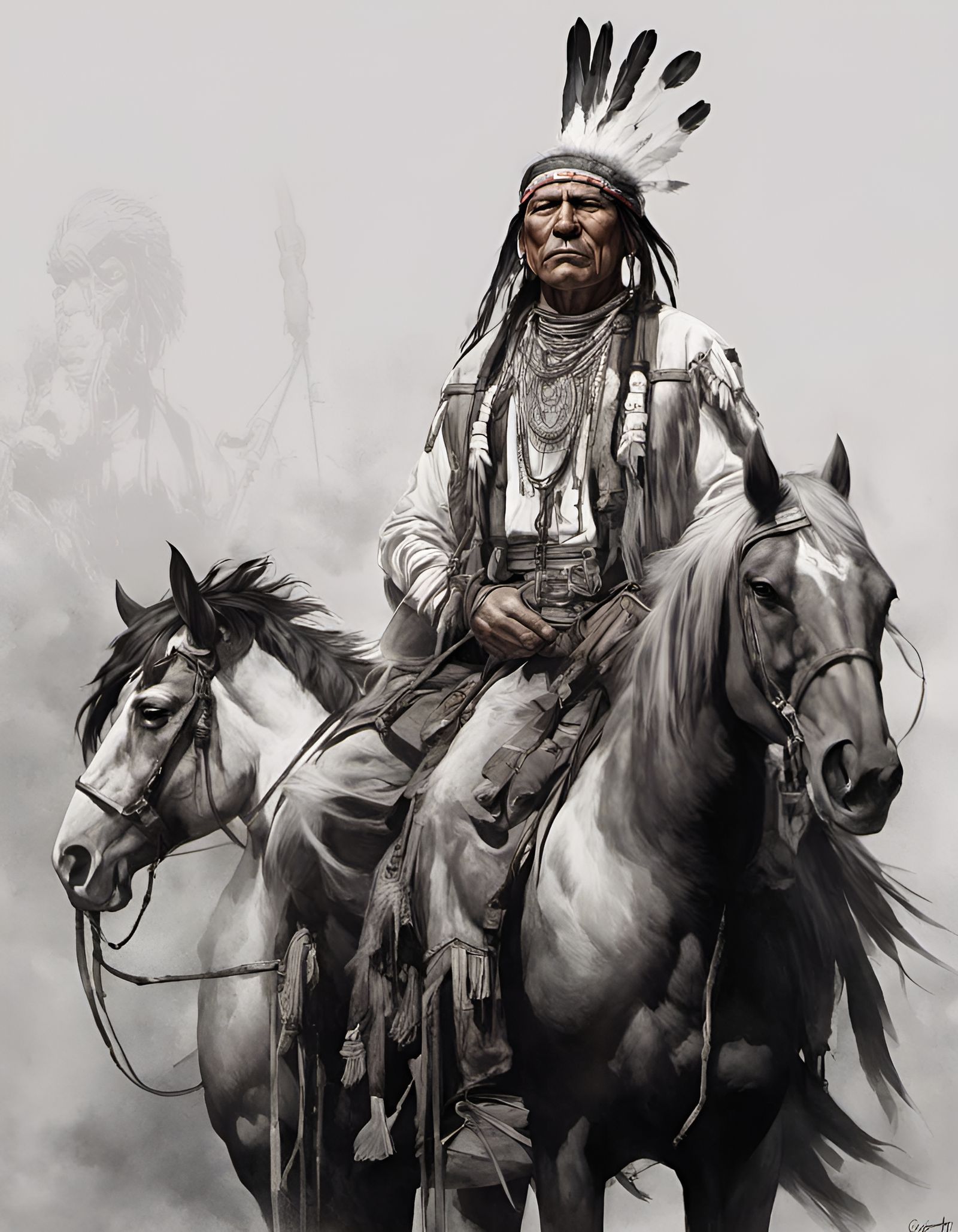The painting depicts an elder Native American man with a tanned, leathery face, sitting side-saddle atop two horses in an intriguing, surreal arrangement. To the left of him, a white horse stands, while on his right a gray horse is positioned, and the man appears to be seated on both their backs. He wears a predominantly white and gray outfit with a black and white tribal headscarf, topped by six or seven feathers. The faint hint of red in his headband provides the only strong color accent in the otherwise muted black, white, and gray palette. His natural brown skin tone adds subtle warmth to the composition. The background, largely white, features the ghostly, incomplete drawing of another Native American to the left, enhancing the ethereal quality of the scene. This unique, almost dreamlike image could be a product of artificial intelligence art, noted for its improbable horse arrangement and old-timey illustration style.